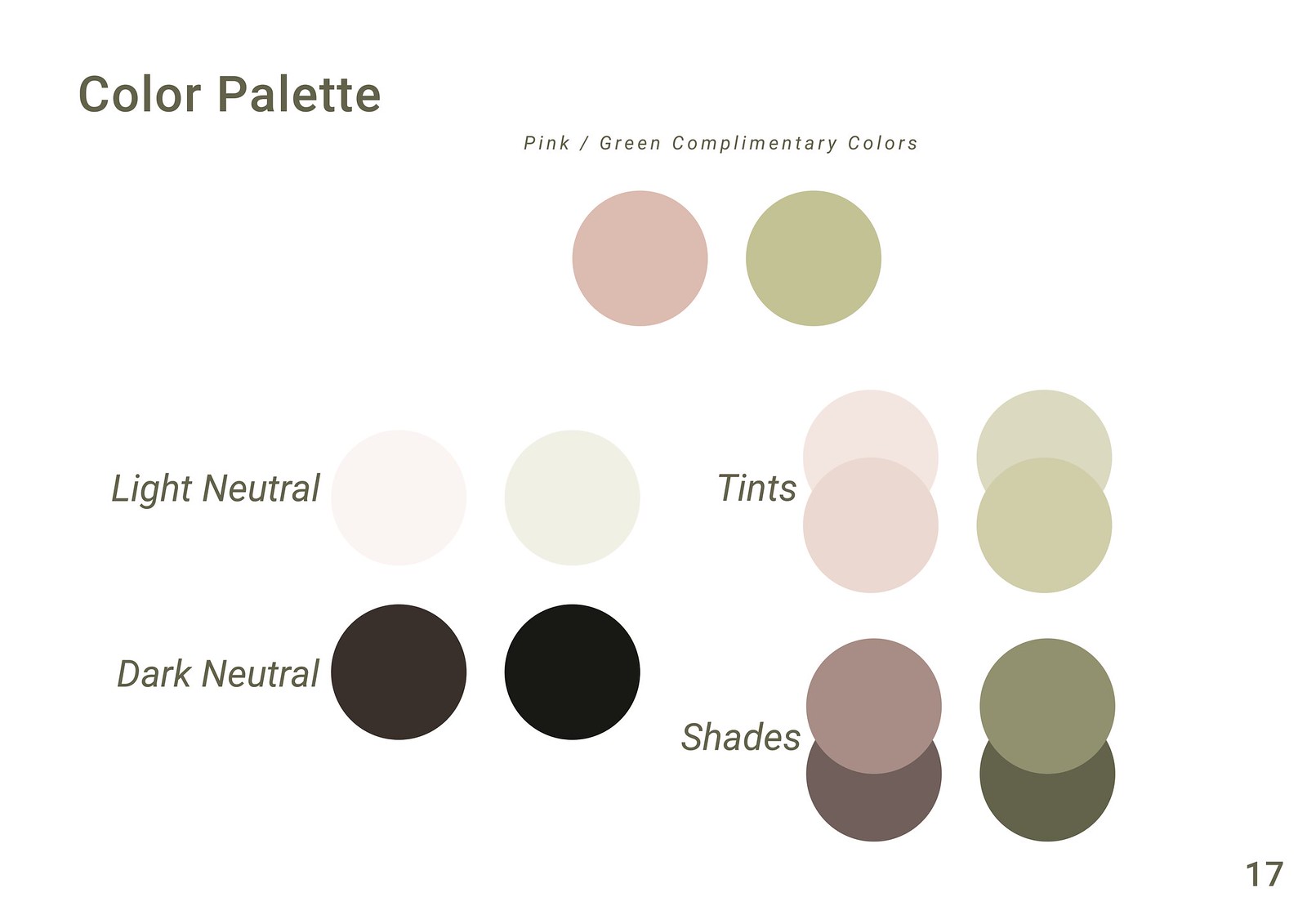The image is a detailed color illustration labeled "Color Palette" at the top left. It features various labeled circles of color arranged in rows. The top row is titled "Pink/Green Complementary Colors" and displays a pink circle next to a green circle. Below that, two columns showcase "Light Neutrals," "Dark Neutrals," "Tints," and "Shades." In the "Light Neutrals" column, there is a light pink circle beside a light green circle. The "Dark Neutrals" column features a dark brown circle and a black circle. The "Tints" section includes a range of hues with a light green circle and a medium green circle stacked next to each other. Finally, the "Shades" section shows a progression from a mauve circle to a dark purple circle and from a sage green circle to a dark green circle. In the bottom right corner, the number "17" is displayed. The overall impression is that these different color groups might represent eyeshadow or makeup palettes.